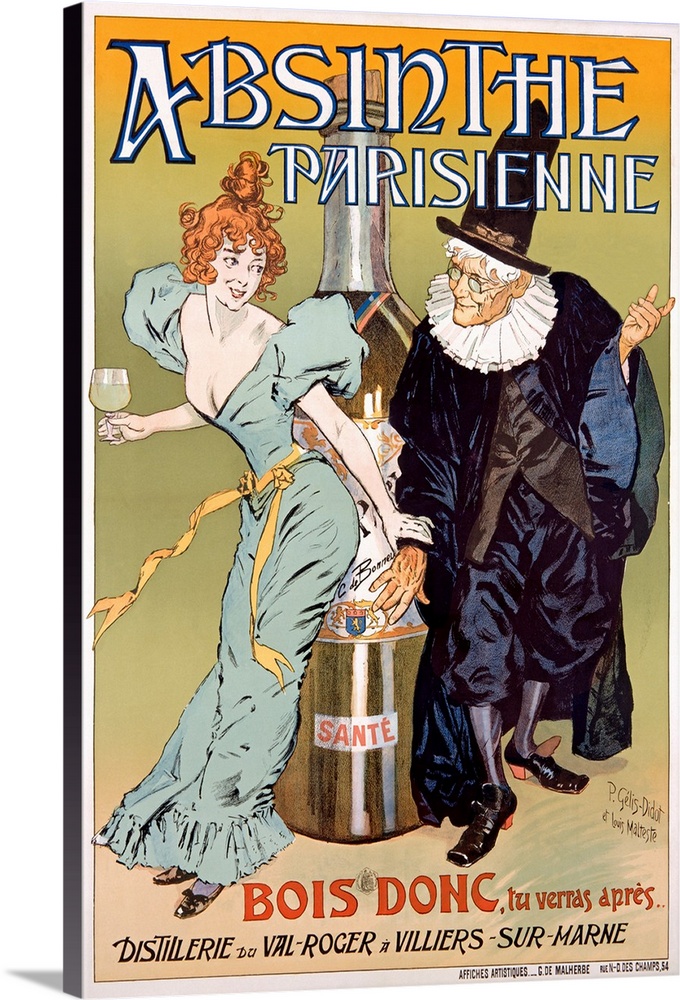This is an artistic book cover with a fairytale-like aesthetic for a title called "Absinthe Parisian." The cover prominently features two characters in a vibrant and stylistic illustration. At the top, the title "Absinthe Parisian" is displayed in bold, white, decorative letters. The background transitions through sunset hues of orange, yellow, and green, down to a dirt-colored base where the characters stand. A red-haired woman with flowing, curly hair is depicted wearing a blue dress with dramatically poofy shoulders and a yellow flowing sash around her waist. Her dress has a deep V-shaped neckline revealing significant cleavage. She is holding a wine glass, presumably with Absinthe, and has one hand placed on a man's arm. The man beside her, characterized as an old wizard-like figure, sports a tall black top hat, gray hair, glasses, and an elaborate black outfit with a furrowed collar. Behind them is an exaggeratedly large bottle of wine labeled "Sante." Underneath the main illustration, various text elements in a different language add to the mystical and foreign allure of the cover, hinting at the book's enigmatic contents with phrases like "Boasdonk Blueberries et Perez."